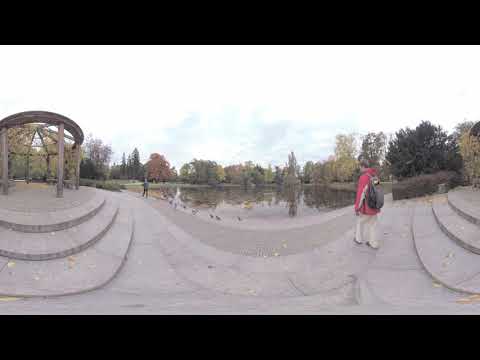In the foreground of the image, a young person in a pink and white striped jacket and white pants stands at the cement border of a man-made lake in a park, gazing at the water. The person, possibly a woman with blonde hair, carries a green backpack. The lake, which has a rectangular shape, is bordered by a walkway that is entirely concrete. 

On either side of the lake, there are curved cement steps leading up to identical gazebos with benches inside; people are seen sitting in these gazebos, one person wearing a gray sweatshirt with a hood and seemingly feeding ducks by the lake's edge. 

In the middle distance, another person in a red jacket and light pants is also visible. Several trees line the lake's far end, meeting a white sky with indistinct clouds and occasional patches of blue. 

The image, taken with a wide-angle lens, shows some distortion, particularly along the bottom portion, giving a concave appearance to the otherwise flat walkway. The overall scene captures a serene moment in a structured yet natural park setting.